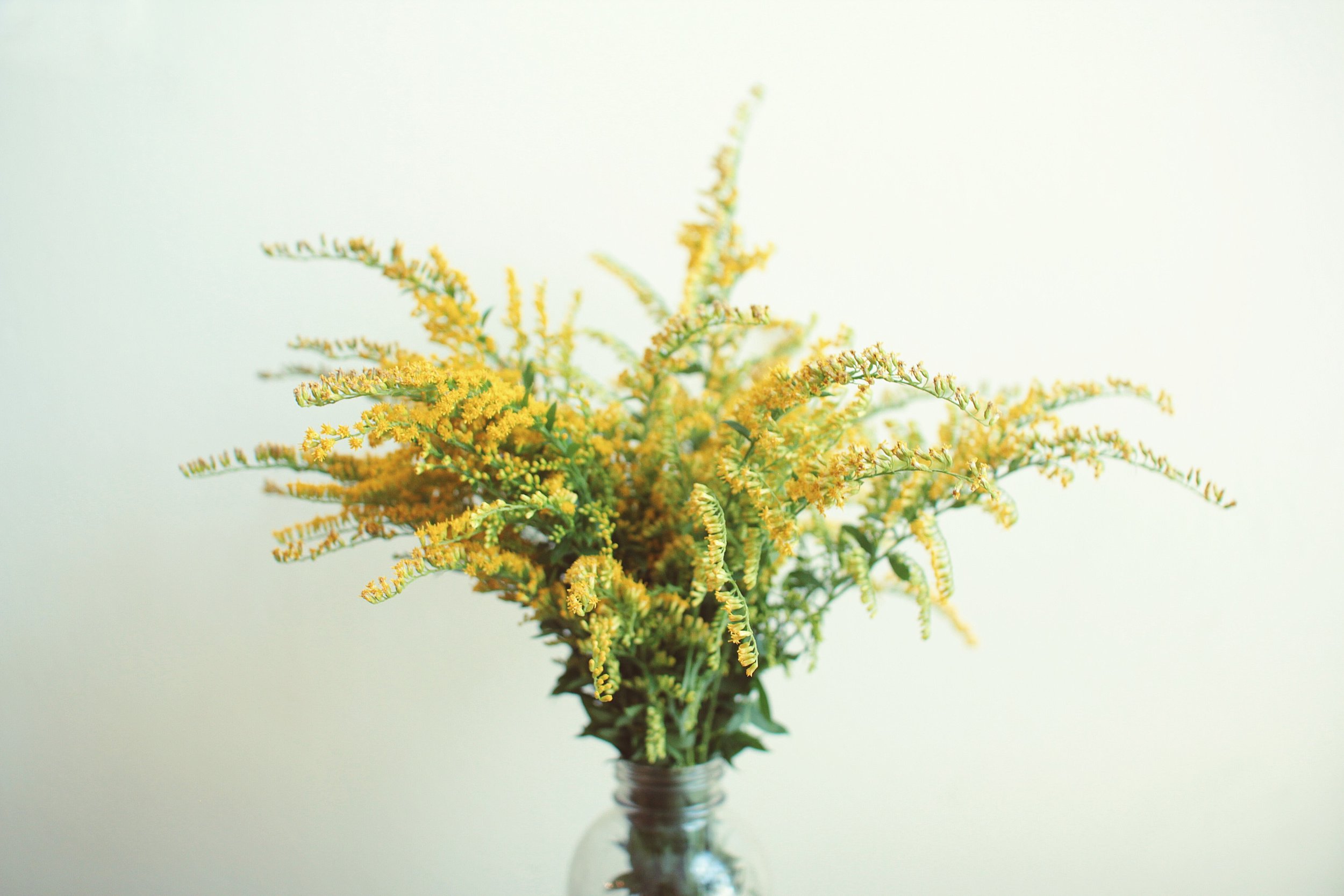The image depicts a minimalist arrangement of yellow wildflowers, reminiscent of goldenrod, centered against a light, almost creamy-colored, possibly light-green backdrop that appears to be softly illuminated, washing out the back right section. The wildflowers, with their delicate, thin green stems and leaves, display clusters of tiny yellow or golden petals. These flowers are tightly bunched together and inserted into a clear glass bottle with a screw-on lid that has been removed, revealing a narrow opening at the top. The bottle itself exhibits a slight glare, reflecting the light softly, and its neck and upper portion are visible, though the contents within it appear just a bit blurry. Shadows cast to the bottom left add depth to this elegant and simple composition.